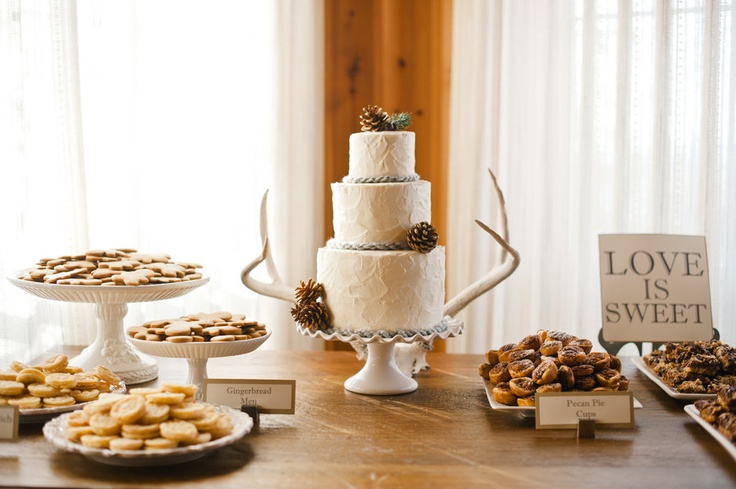In the center of the photograph, a striking three-tiered white wedding cake stands poised on a white riser atop a rustic brown wooden table. The cake is adorned with pinecones and flanked by antlers, lending a natural, woodland touch. To the left, there are plates filled with assorted cookies, including gingerbread men on white risers, with a coordinating sign. On the right side, a plate of pecan pie cups is similarly labeled, with an additional sign in the back proclaiming "LOVE IS SWEET" in bold capitals. The background features white curtains over windows and wood paneling directly behind the cake, framing the delectable display of sweet treats.